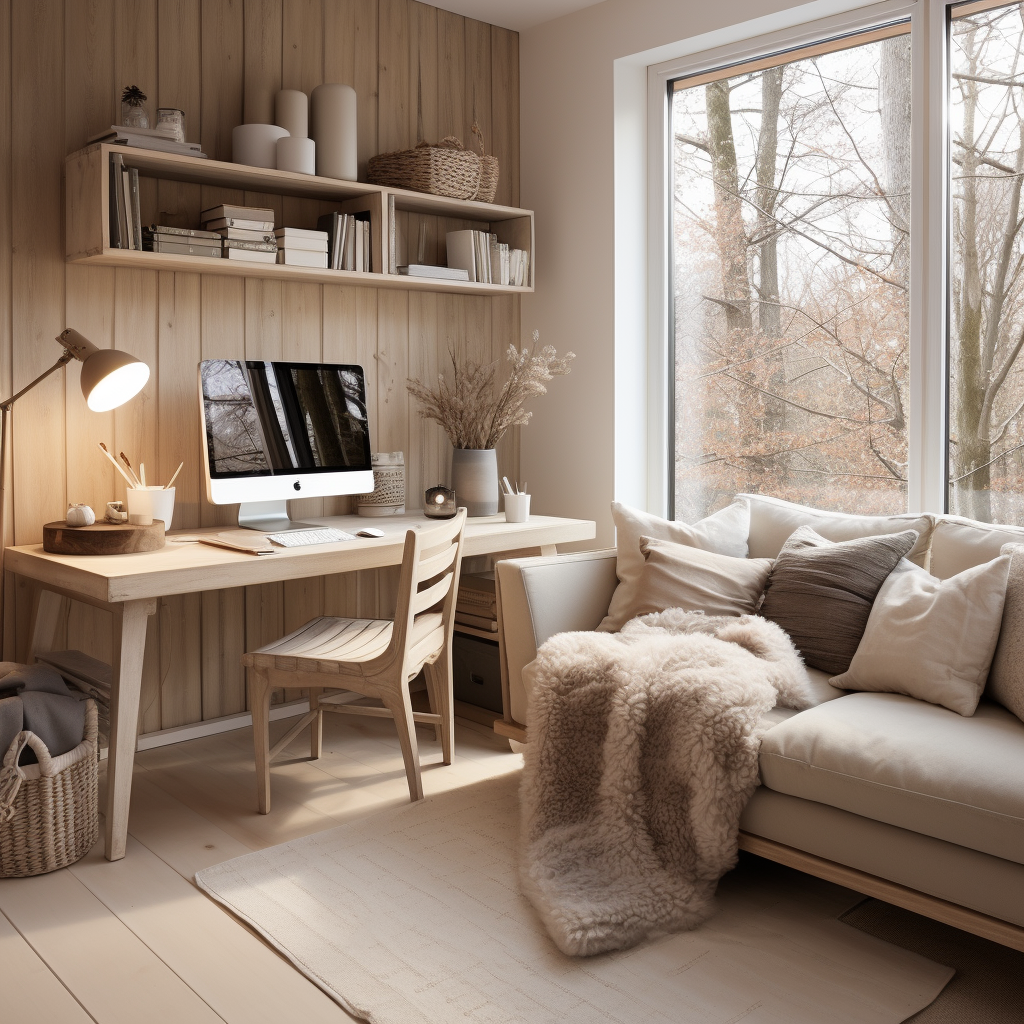The image depicts a meticulously organized workspace, evoking a nearly AI-generated aesthetic, albeit with slightly pixelated details. On the left side of the wooden desk rests an Apple iPhone, its screen illuminated. Scattered across the desk are several pins, adding a touch of casual clutter. Mounted above the desk are two square shelves, each neatly filled with an assortment of books. Various tools are arranged at the top, suggesting a multi-functional workspace. Adding a touch of nature, a thriving plant in a vase sits prominently on the desk. The setup also includes a sleek keyboard and a mouse, highlighting the desk's functionality. To the right of the desk, a cozy couch invites relaxation, while the floor below is visible, grounding the scene. The ceiling is adorned with warm brown tiles, enhancing the autumnal atmosphere indicated by the fall season. Overall, the scene captures a harmonious blend of productivity and comfort.